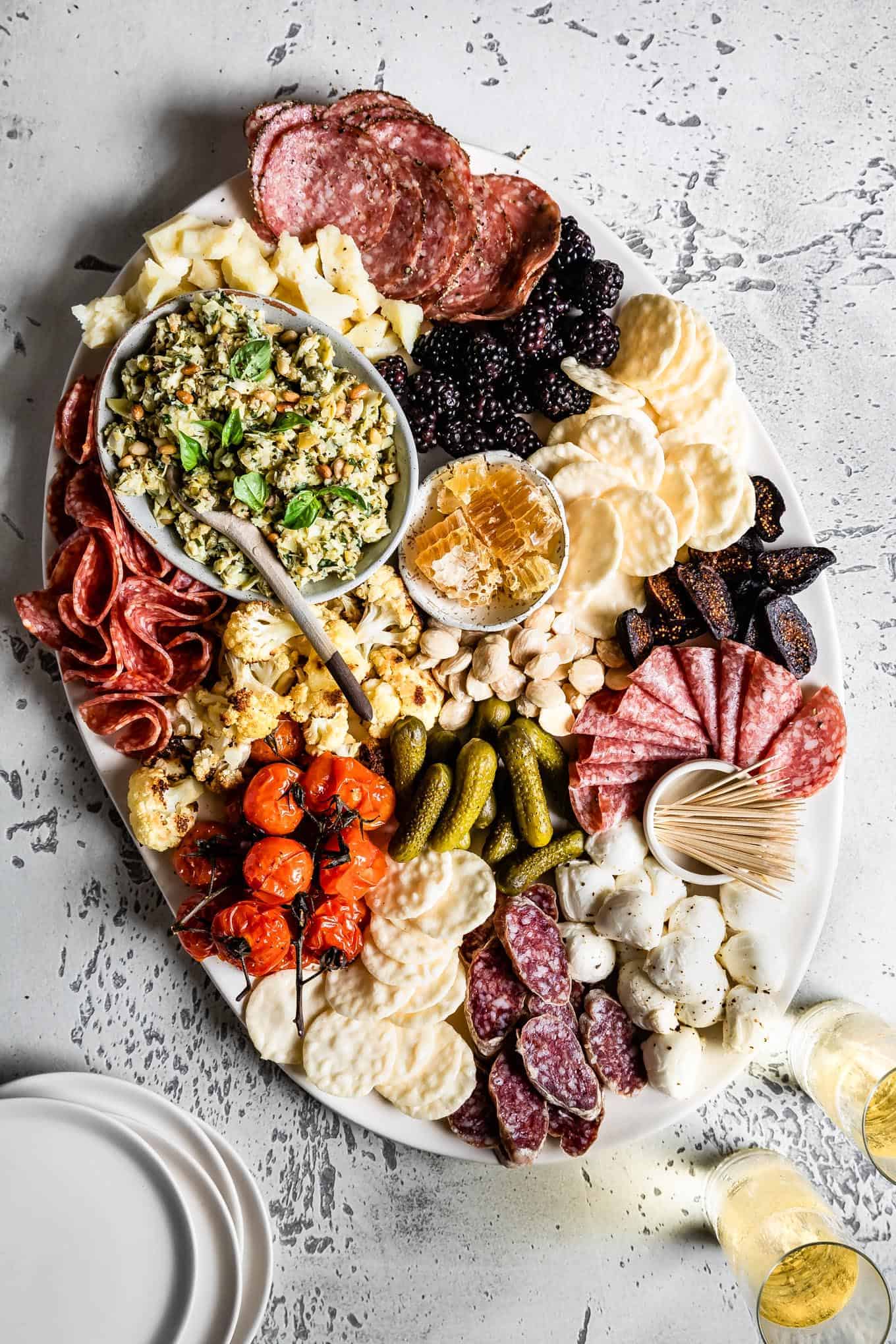This vertical rectangular color photograph showcases an elaborate charcuterie platter displayed on a white and black etched marble surface. The large, white, oval platter is brimming with an assortment of foods, all artfully arranged and touching, creating a visual feast. 

Key items on the platter include at least four types of salami, dark-colored sausages sliced into rounds and formed into cones, and white crackers interspersed throughout. Small bocconcini and mozzarella pearls are dotted around, adding a soft, white contrast to the meats. Bright pops of color come from blackberries, roasted tomatoes on vines, gherkins, and roasted cauliflower. In the center is a small bowl with honeycomb and white cheese, adding an element of sweetness.

Adjacent to the platter, on the bottom left, is a stack of circular white plates ready for serving, while the bottom right features two champagne flutes filled with light yellow liquid. A bowl with salad, accompanied by a wooden spoon, is positioned next to another dish holding toothpicks for easy self-service. Nearby, a glass of wine is stationed next to a bowl that completes this sumptuous spread. The entire setting conveys an inviting and somewhat challenging assortment, perfect for a grand culinary experience.